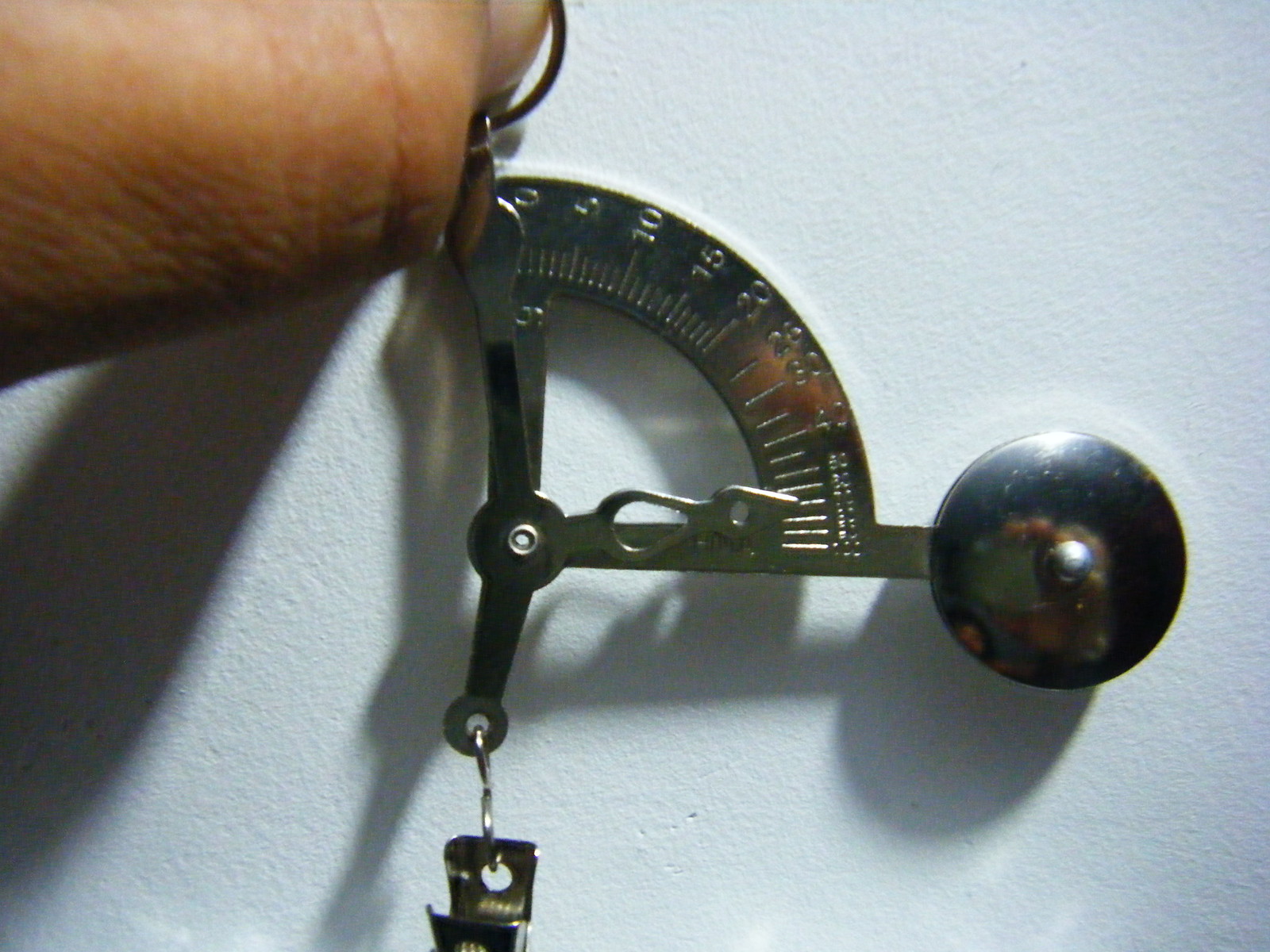The image depicts a metal measuring device positioned on a white surface, with part of a human hand visible in the top left corner holding the device. The device features a quarter-circle scale on its left side, marked with increments from 0 to 40, at intervals of 5 units. Numerous smaller lines for finer measurements are also visible along this scale. A horizontal support bar runs beneath the quarter-circle scale, extending to a circular metal disc on its right side. The device, resembling a protractor or an angular measurement tool, appears to have a slightly tarnished silver or brass finish. Additionally, there is an element hanging from the bottom of the device by a hook, possibly a clip. The background is entirely white, emphasizing the detail and structure of the measuring tool.